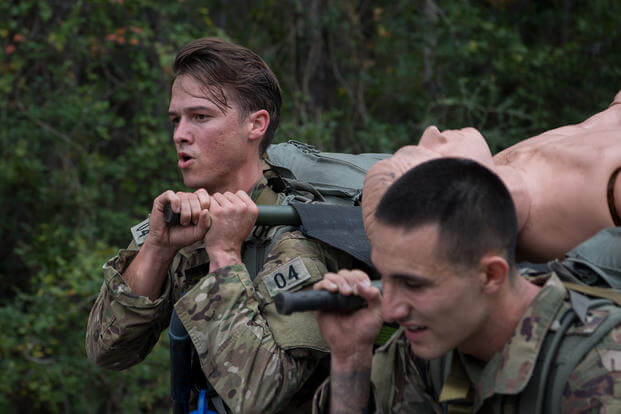In a dense, green, forested setting, two young soldiers are diligently engaged in a training exercise. Both are clad in fatigues—a mix of brown, tan, and green camouflage patterns. The soldier closer to the camera, positioned at the bottom right, has a shaved black head and appears focused as he grips the front handle of a canvas stretcher. His fellow soldier, positioned to the left and further in the background, sports medium-length dark hair, contrasting with the typically shaved look seen in training environments. He also bears a visible number "04" on his sleeve and handles the opposite end of the stretcher. Together, they carry a plastic, skin-colored dummy on the stretcher, simulating a scenario that tests their endurance and teamwork. Both soldiers look visibly tired, highlighting the strenuous nature of their task. The absence of distinguishing features or packs suggests that the emphasis here is on mastering the carrying technique and coordination under the canopy of lush, green trees that enclose the training area.